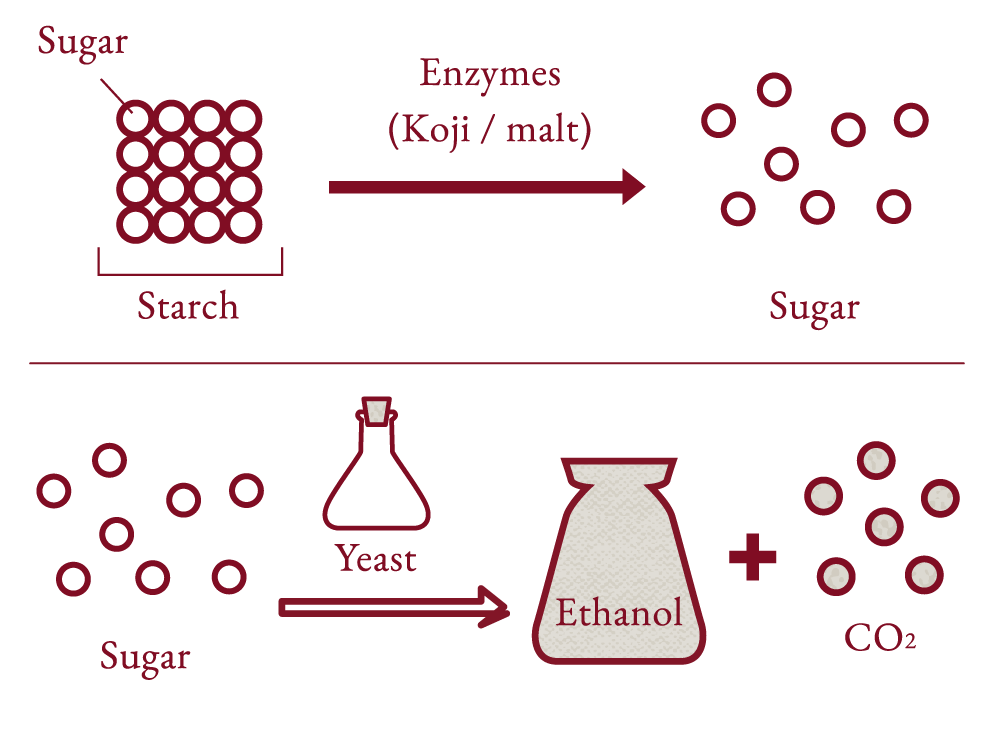The image is a hand-drawn scientific diagram on a white background, divided by a red horizontal line at its center. The top half of the diagram illustrates the conversion of starch into sugar through enzymatic action. In the top left, a grid of sixteen red circles (arranged in a 4x4 pattern) is labeled "starch," with an arrow pointing from one of the circles towards a text indicating the presence of enzymes (specified as "koji/malt"). On the right side of this section, there are eight smaller, individual red circles labeled "sugar," showcasing the breakdown process.

The bottom half of the diagram demonstrates the conversion of sugar by yeast into ethanol and carbon dioxide. Scattered red circles, representing sugar, are shown on the left side. There are labeled bottles of yeast and ethanol, with "CO2" and "ethanol" highlighted and filled in gray, indicating the byproducts of the reaction. The diagram effectively breaks down the steps of transforming starch into sugar, and subsequently converting sugar into ethanol and CO2, with a clear and simplistic visual style that enhances understanding.